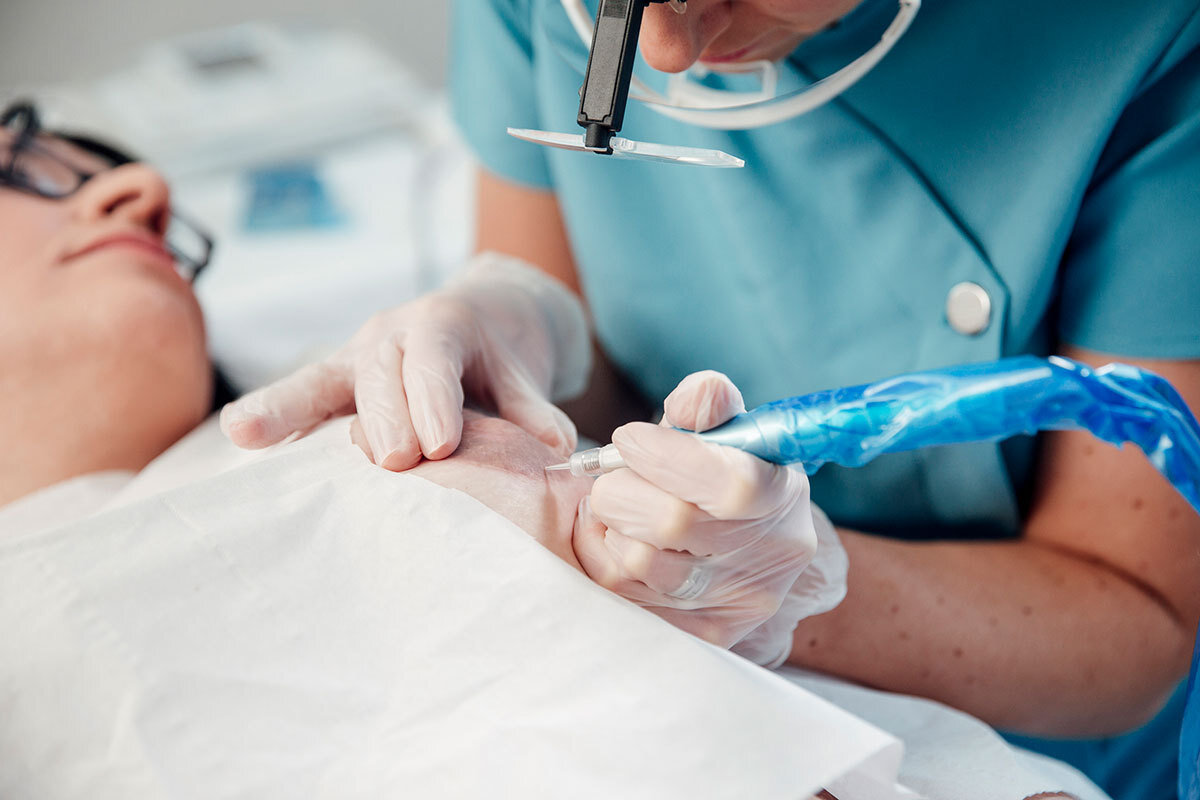This detailed image captures a medical professional, potentially a doctor, attending to a patient in what could be a medical office or a tattoo parlor. The patient, whose gender is indeterminate due to the close-up nature of the photograph, is lying down wearing a white protective bib and wire-rimmed glasses. The focus of the image is the patient's upper body, particularly an area that could be the arm, shoulder, or nipple, which the professional is working on.

The medical professional, who has pale, freckled skin and is attired in blue scrubs with metallic round buttons, is wearing white plastic surgical gloves. They are holding a pen-like device with a blue handle in their left hand, which looks like a needle or possibly a tool used for either tattooing or a medical procedure, such as mole removal or injecting medication. The device appears to be applied to the patient's skin, suggesting a precise and delicate procedure.

Additionally, the medical worker is equipped with headgear that includes safety goggles and a magnifying lens, presumably to enhance their view of the work area. The background of the image remains blurred, ensuring that the primary focus remains on the interaction between the healthcare professional and the patient, highlighting the intricacies of the procedure being performed.